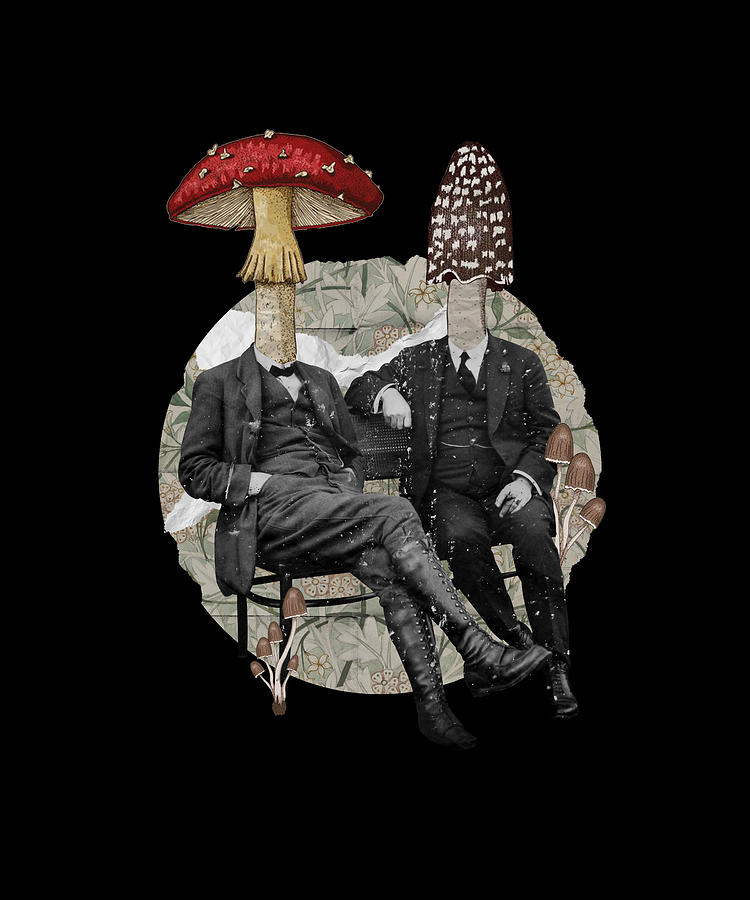This image depicts a surreal, modern art piece set against an all-black background. At the center is a rounded, padded futon chair adorned with a floral pattern in shades of green and faint reds. Seated on this chair are two gentlemen dressed in three-piece vintage suits, complete with white shirts and ties. The man on the left sports black knee-high leather boots with his pants tucked into them and a red mushroom with white spots for a head. His right hand is in his pocket, and his left hand also seems to be in his pocket. The man on the right, who is wearing dress shoes and also has his right arm draped over the back of the chair, has a brown mushroom with white spots for a head. Both men's faces have been replaced by these large, colorful mushrooms, giving the piece its surreal quality. Surrounding them are smaller mushrooms with brown caps and white stems, subtly integrating them into the chair’s floral pattern. The background also features a circular fabric with crinkled textures in khaki, tan, and ecru, adding to the artwork's intricate details and depth.